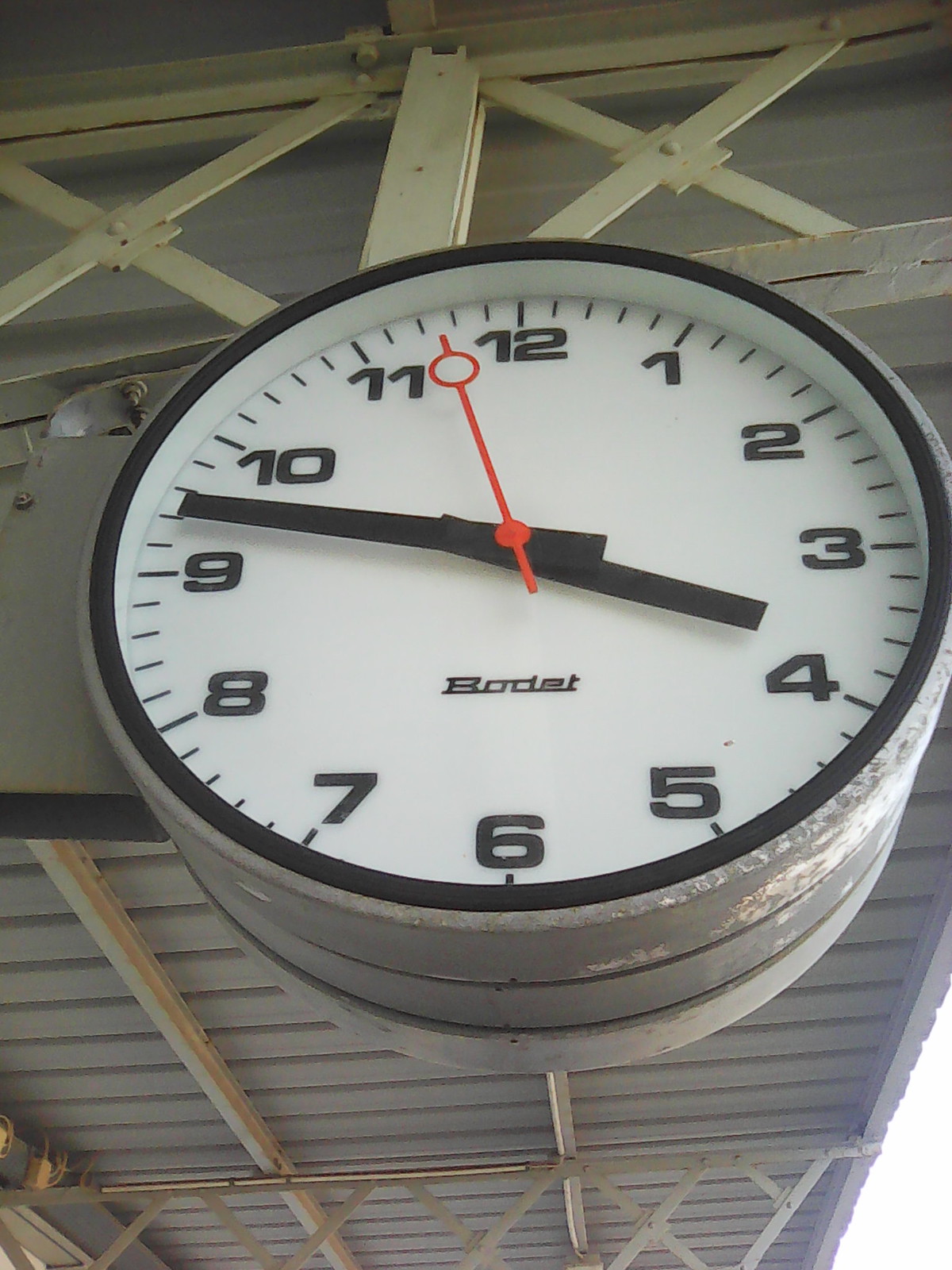In this color photograph, we observe a large, circular clock hanging from the steel rafters of a high, metal-ceilinged structure, possibly a train station or sports stadium. The rafters are painted yellow, contrasting with the gray, tarnished yet unrusted metal of the clock's barrel-shaped exterior, which measures about half a foot in thickness. The clock’s face is stark white, encircled by a plain black rim, and features black hour and minute markers with large black numerals. The minute hand points between 9:42 and 9:43, while the hour hand is close to the 4, and the red second hand hovers between 11:57 and 11:58. Notably, the clock displays "BODET" in black lettering beneath the hands. The clock's design indicates it may be double-faced, allowing visibility from either side of the building.